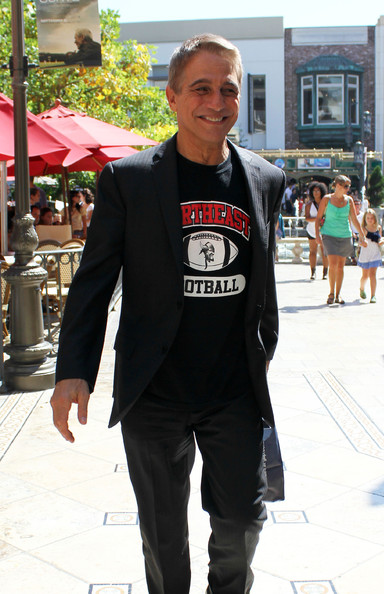This photo features actor Tony Danza strolling along a sunlit sidewalk, smiling directly at the camera. He is dressed in a dark pinstripe sport coat paired with dark slacks and a crew neck t-shirt that reads "Northeast Football" in red text, partially covered by his blazer. The shirt also features a black and white football graphic. Behind him, there's a vibrant street scene that appears to be part of a shopping center or outdoor mall. To the right, a dark green lamp post stands tall, while further back, red umbrellas cover a seating area reminiscent of an outdoor café. Additional background elements include various buildings and storefronts. In the scene, a woman in a skirt and tank top is visible holding a young girl's hand, with another woman casually walking further behind. The overall setting suggests a bustling, communal outdoor space, captured beautifully on a bright sunny day.